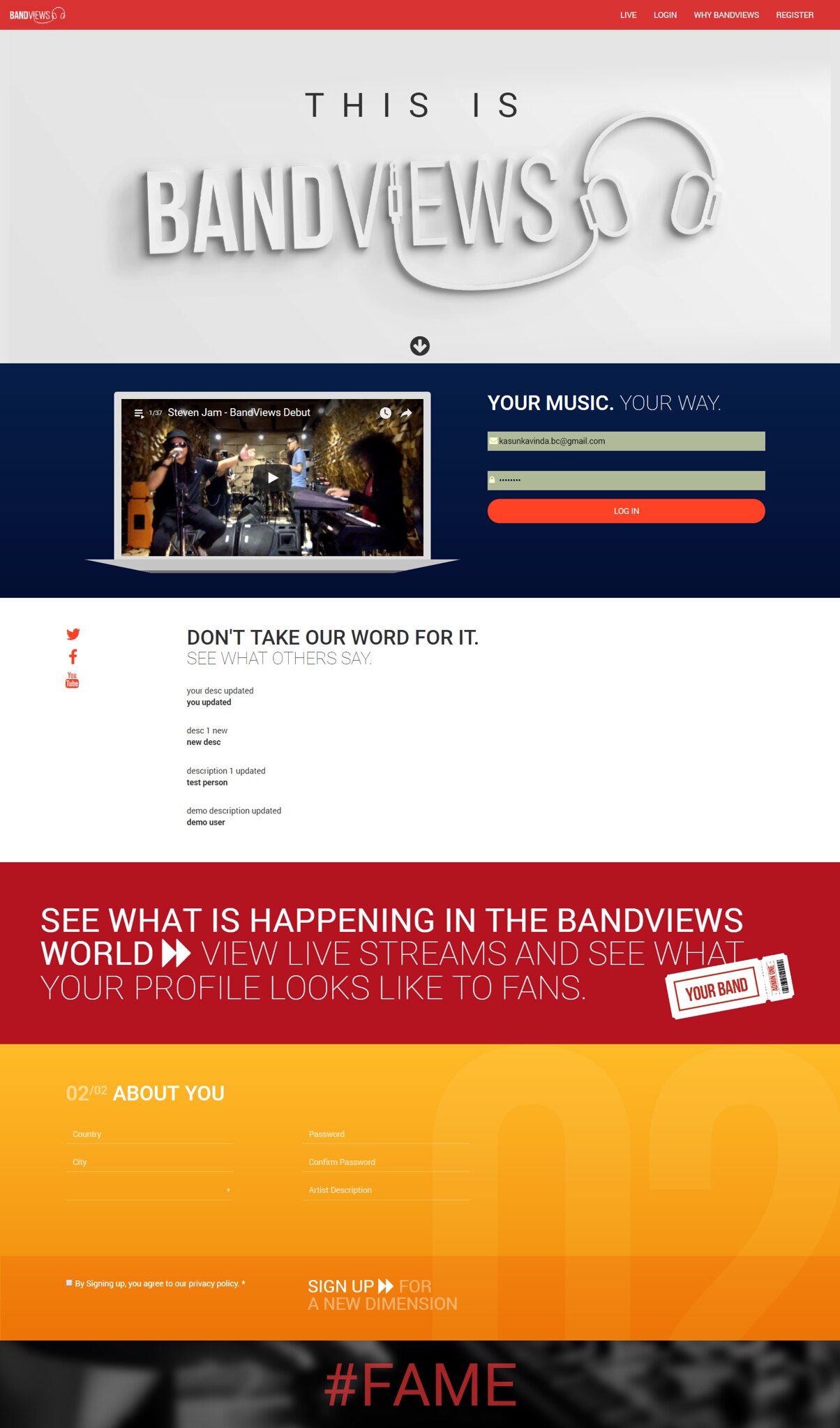The image depicts a computer-generated advertisement for a music service called "BandViews," featuring both text and a small picture of a man performing at a piano. At the top of the image, a white banner with the text "This is BandViews" is prominently displayed, with the "I" in "views" cleverly designed as the plug of a pair of headphones, which extends to show the headphones themselves. Below this, on a blue background, there's a small, somewhat unclear image resembling a YouTube screenshot that likely shows the man playing the piano, accompanied by a play button indicating it is a video.

The central message, written in white on the blue background, reads "Your music, your way," followed by a space for users to enter their username and password, alongside an orange "Log In" button. Another key phrase, "Don't take our word for it, see what others say," encourages users to trust peer reviews. Further down, a wide red banner informs viewers to "See what is happening in the BandViews world, view live streams and see what your profile looks like to fans." Finally, at the bottom of the image displayed on a black background with red lettering, the text reads "#FAME" in all capital letters. The color scheme throughout the image includes black, white, blue, brown, red, yellow, and orange, with black and white used variably in the text. The overall serious and promotional style effectively aims to engage musicians to sign up and participate in the BandViews service.